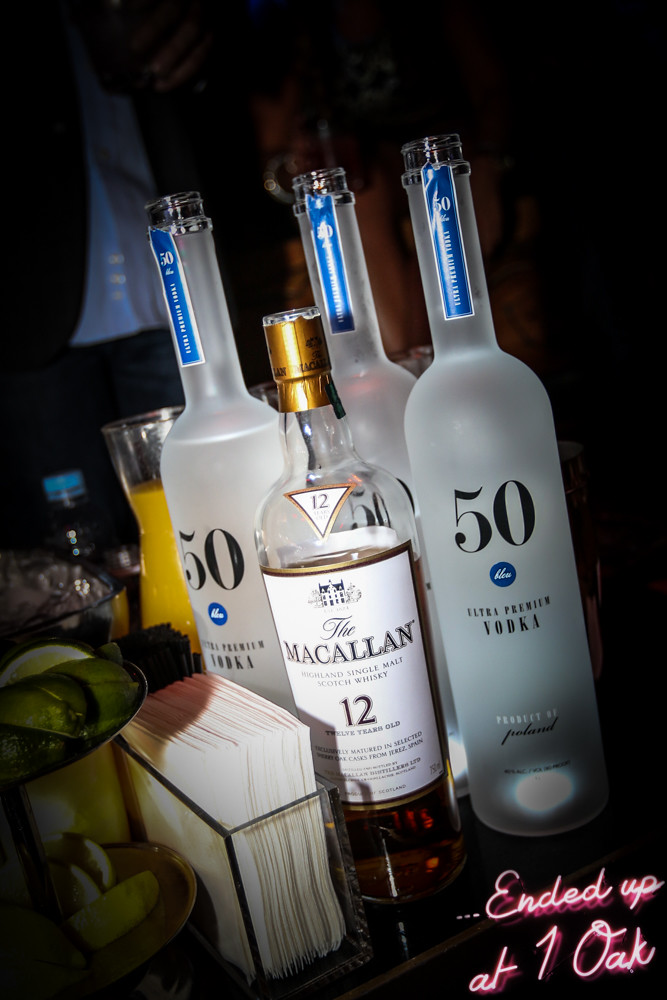In this detailed image, taken at some kind of event, several vodka bottles are prominently displayed on a glass countertop with wood sides. The forefront features three identical bottles of 50 Ultra Premium Vodka, distinguished by their frosted white glass and black text. These bottles have visible, torn stickers indicating they've been opened. Centered among them is a shorter bottle of Macallan Highland Single Malt Scotch Whisky, aged 12 years, adorned with gold accents and partially filled with amber liquid. To the left of the bottles sits a square napkin holder filled with white napkins. Behind this arrangement is a vase-like pitcher filled with orange juice. The background of the image is predominantly dark, adding contrast to the vibrant elements in the foreground. In the bottom right corner, the words "Ended Up at One Oak" are displayed in a neon lighting style, enhancing the event-like atmosphere of the scene.